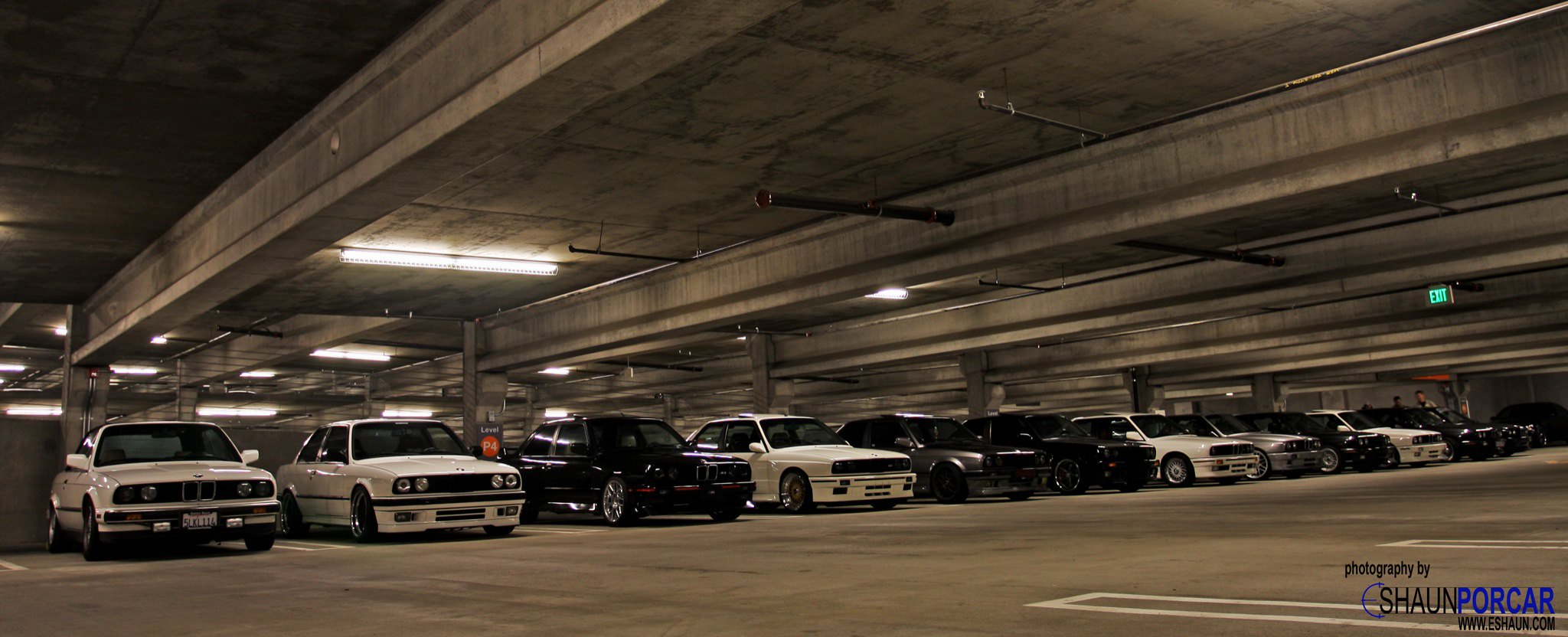This is a detailed photograph of a dimly lit underground parking garage. All the cars are backed into their spaces, with the fronts facing the camera. The garage has a light gray cement pavement marked with white boundary lines for each parking space. The solid gray cement ceiling above is adorned with several large, thick support beams, black pipes, and occasional LED lights. The image, taken from an angle that emphasizes the extreme perspective of the ceiling, also features a lit green exit sign positioned in the middle right of the frame. In the distant background, more lights from the ceiling are visible, adding depth to the scene. The bottom right corner of the photograph bears the text, "Photography by Sean Porcar," with Sean's name spelled as S-H-A-U-N P-O-R-C-A-R, and some smaller, unreadable text below.